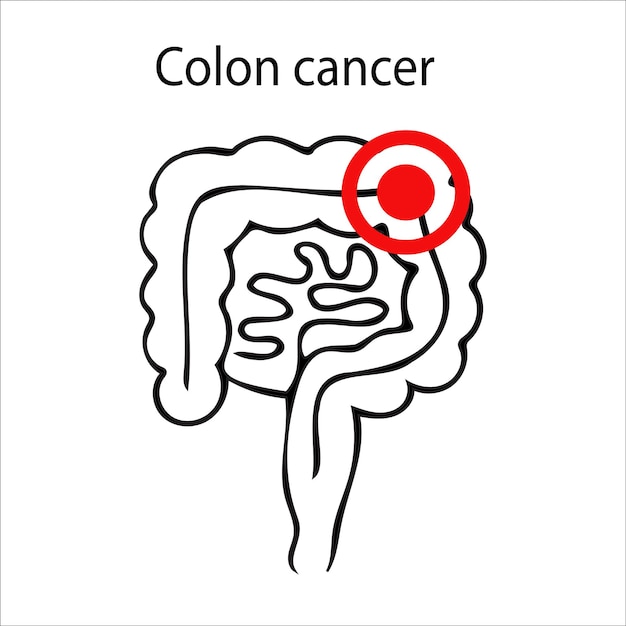The image is a very basic, black-and-white medical diagram labeled "colon cancer" at the top. It depicts a simplified representation of the large intestine with minimal complexity and detail, displayed against a plain white background. A red dot enclosed in a red circle marks the upper right area of the intestine, indicating the location of the cancer. The surroundings of the intestine, which could represent the stomach or the small intestine, are indistinct. The overall low-quality and straightforward design of the image resembles something one might find on a basic medical document or an educational website like Wikipedia.